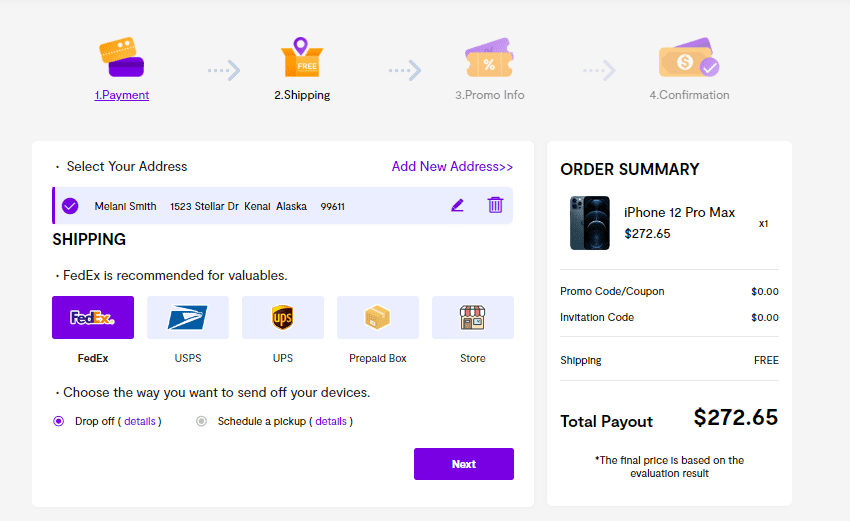The screen capture displays a webpage for an order process. The background is gray, and across the top are four icons illustrating the order progression. From left to right, the icons are labeled: "Payment," "Shipping," "Promo Information," and "Confirmation." The "Payment" icon is highlighted, indicating completion, while the current step is "Shipping."

In the lower half of the image on the left, there is a section for address selection. It includes options to "Select Your Address" or "Add New Address." Below these options, the selected shipping address is displayed: "Malia Smith, 152 Stellar Drive, KENAI, Alaska 99611." The section continues with a note recommending FedEx for valuables and lists various shipping options: FedEx, UPS, Prepaid Box, and Store.

At the bottom, users can choose their shipping method with options like "Drop Off" and "Schedule a Pickup."

On the right side of the screen is the order summary. It shows an "iPhone 12 Pro Max" priced at $272.65. No values are entered for the "Promo Code" or "Invitation Code." Shipping is listed as free, bringing the total payout to $272.65.